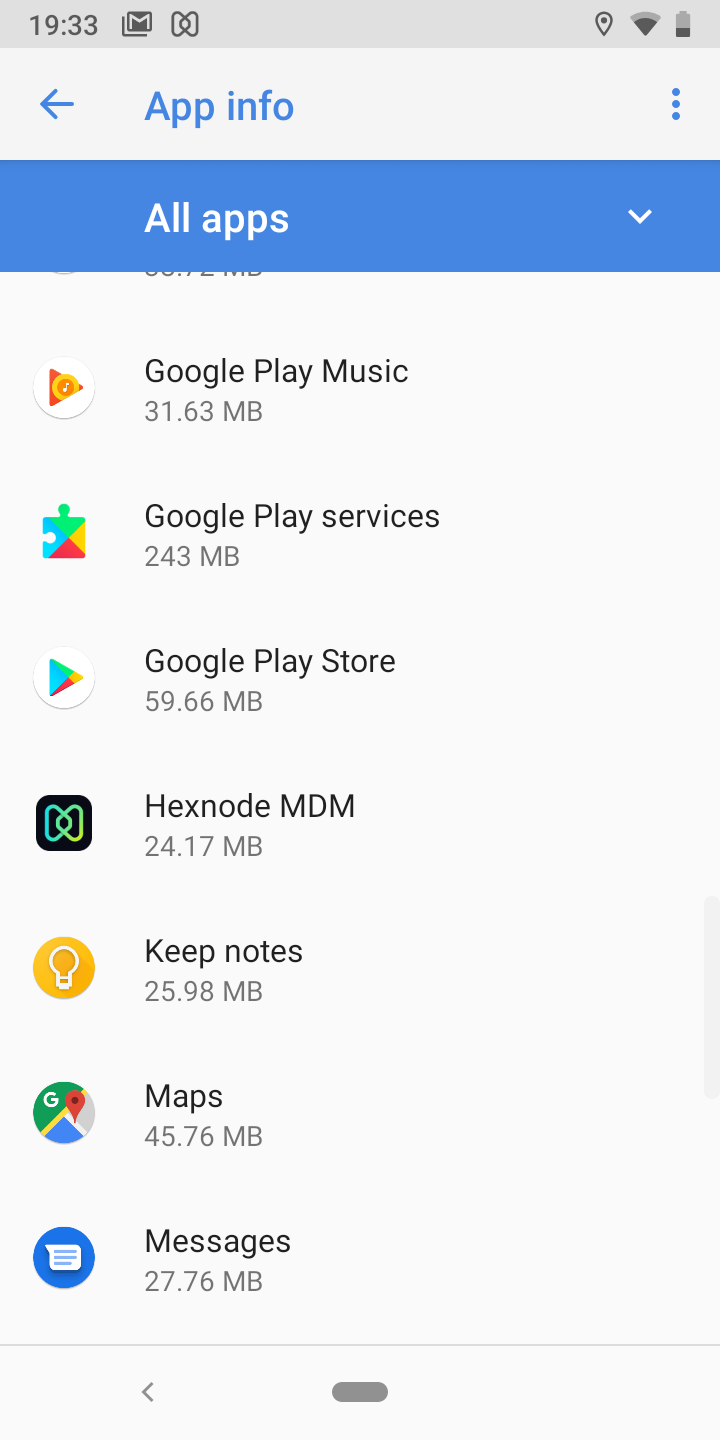This is a detailed screenshot of a mobile phone displaying a list of applications. At the top, the header is a medium gray color. In the top-left corner, in gray text, is the time "19:33." To the right of the time, there is a Gmail icon. Next to it, there's an icon made up of two triangles with rounded corners and wide bases facing left and right, respectively. Further to the right, a geolocation pin icon is displayed. Adjacent to this, there is a Wi-Fi logo showing a signal strength of about two-thirds. Finally, in the top-right corner, a battery symbol is visible, indicating a charge level of about a quarter full.

Beneath this header, the bulk of the screen has a light gray background. At the top of this area, a blue header reads "App Info," accompanied by a blue arrow pointing left. On the right side of this header, there are three vertically arranged blue dots. Below, a medium blue bar spans across the screen with white text that reads "All Apps," and a white arrow pointing downward is positioned on the right side of this bar.

The main section of the screen lists seven applications vertically, each with its icon and the amount of storage space it occupies:
1. **Google Play Music** – 31.63 MB
2. **Google Play Services** – 243 MB
3. **Google Play Store** – 59.66 MB
4. **Hexnode MDM** – 24.17 MB
5. **Notes** – 25.98 MB
6. **Maps** – 45.76 MB
7. **Messages** – 27.76 MB